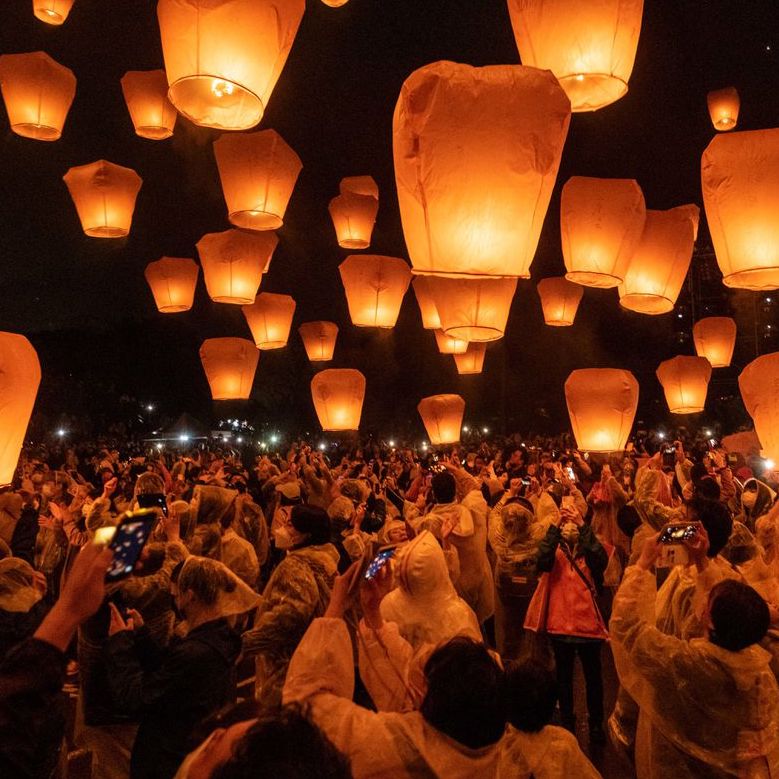This color photograph captures a large nighttime gathering of hundreds of people, all bathed in a warm orange and yellow glow cast by numerous illuminated paper lanterns suspended above their heads. The sky is pitch black, providing a stark contrast to the radiant lanterns, which are likely lit by candles, giving off a soft, ethereal light that floods the scene with a warm hue. Dressed in various outfits, many attendees wear raincoats or parkas, suggesting it might be raining. Virtually everyone in the crowd is holding up a smartphone to capture this mesmerizing view. The contrast of glowing lanterns and the sea of people, each contributing to the splendor with countless tiny white dots from their phone screens, creates a vibrant and dynamic atmosphere.